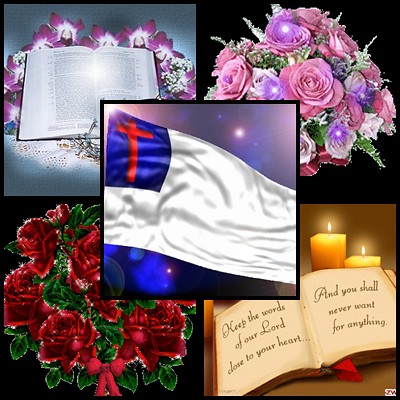The image is a Christian-inspired card featuring a collage of five distinct square photos. The upper left quadrant displays an open Bible adorned with flowers. Adjacent to it, in the upper right quadrant, sits a beautiful bouquet of mixed-color flowers, including purple and red. Below this, in the lower right quadrant, another open book, possibly a psalm book, is shown with lit candles behind it. The caption around this book reads, "Keep the words of our Lord close to your heart and ye shall never want for anything." In the lower left quadrant, there is a bouquet of red flowers with green leaves. At the center of the composition is a superimposed Christian flag featuring a white background, a blue canton, and a red cross. The scene aims to inspire with a serene and reverent motif. Additionally, there seems to be the initials "ZW" subtly placed in the lower right corner beneath the book.